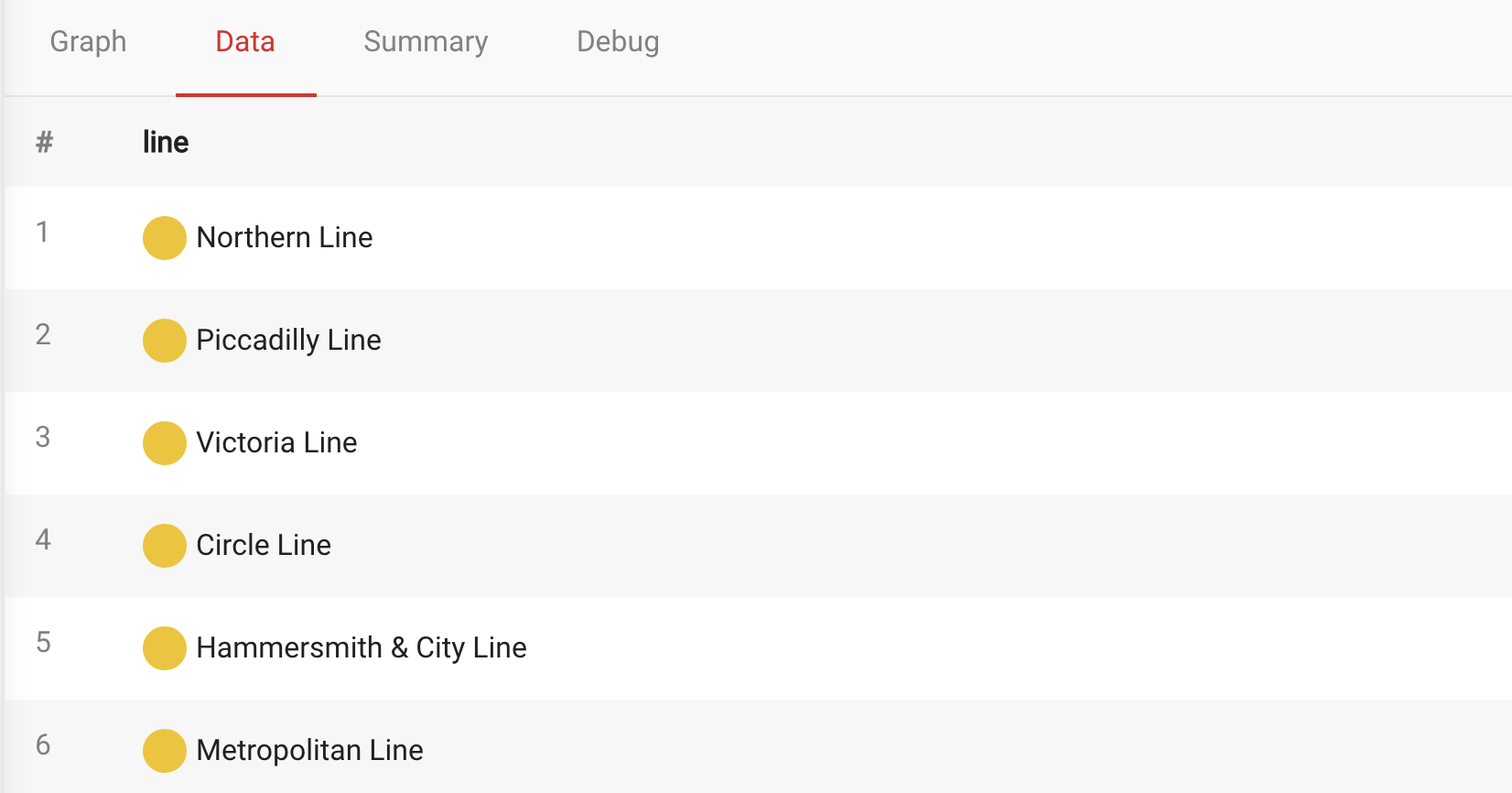In the image, there is a list of subway lines with detailed categorization and formatting. On the top left corner, four categories are displayed: "Graph," "Data," "Summary," and "Debug." The categories "Graph," "Summary," and "Debug" are all in gray, whereas "Data" is in red and underlined, indicating it is the selected category.

The list of line names is organized in a column, with alternating gray and white backgrounds for each row, creating a visually distinct separation between the entries. Each line name is preceded by a yellow circle and a line number. The line numbers and names are as follows:
1. Northern line
2. Piccadilly line
3. Victoria line
4. Circle line
5. Hammersmith and City line
6. Metropolitan line

All the line names are written in black, providing clear readability against the alternating background colors. This organized and color-coded layout facilitates easy navigation and selection within the categorized data.